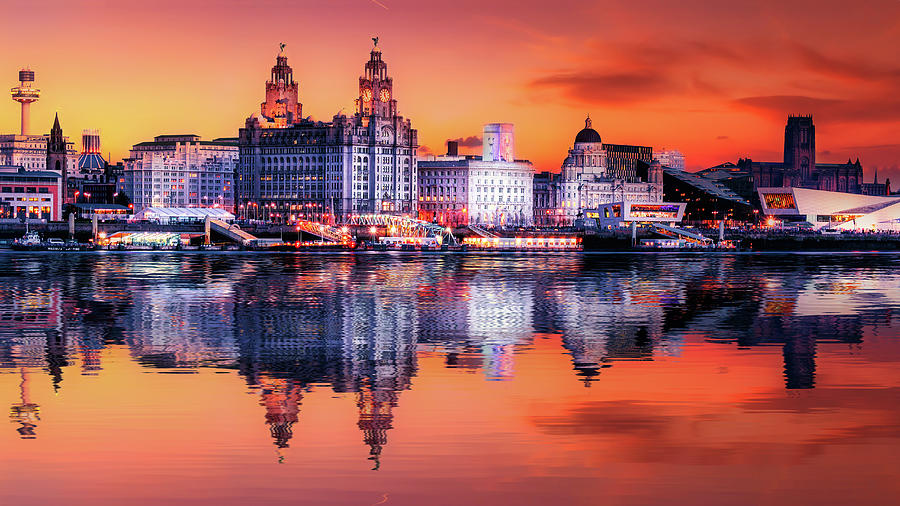This photograph captures the enchanting view of a historic European city, possibly resembling Oslo or a Swedish city, as seen from across a serene river. Taken during late sunset, the sky is a vibrant gradient of yellow to deep orange, reds, and purples, casting a fiery glow that reflects on the still waters below. The city's waterfront is alive with lights, adding a warm ambiance to the scene. The cityscape features a harmonious blend of old and new architecture: majestic gothic cathedrals with steeples and clock towers, classical masonry buildings, contemporary structures with distinctive slanted roofs, and a modern museum along the riverbank. Domes and spires punctuate the skyline, which is mirrored perfectly in the tranquil river, creating a symmetrical and picturesque reflection. The overall composition of the photograph elegantly balances the luminous evening sky, the historic and modern structures, and their captivating reflections in the water.